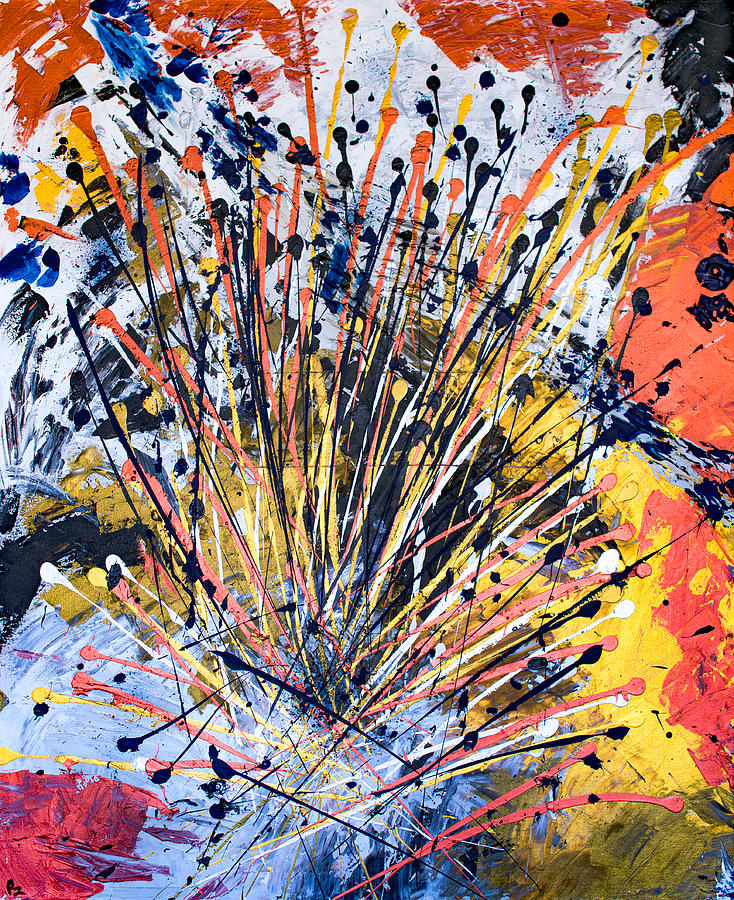This image displays a vertically-oriented, square painting reminiscent of Jackson Pollock’s iconic style. The canvas is a chaotic riot of colors featuring drips, splatters, and streaks of paint in black, white, orange, yellow, red, and a hint of blue. The white of the canvas peeks through in places, adding to the overall tumultuous feel. Paint is applied in seemingly random directions, creating a sense of frenetic energy without any discernible pattern or figure. Prominently within the center, various colors—predominantly black, orange, yellow, and white—dominate the scene, while the rest of the canvas carries smears and drips of the same hues intermingled with blue. The lower right corner of the painting discreetly features the mark "P2," possibly the artist's signature or a notation, further adding an element of intrigue to the art piece. The overall effect is a visually compelling and deliberately chaotic abstract composition.